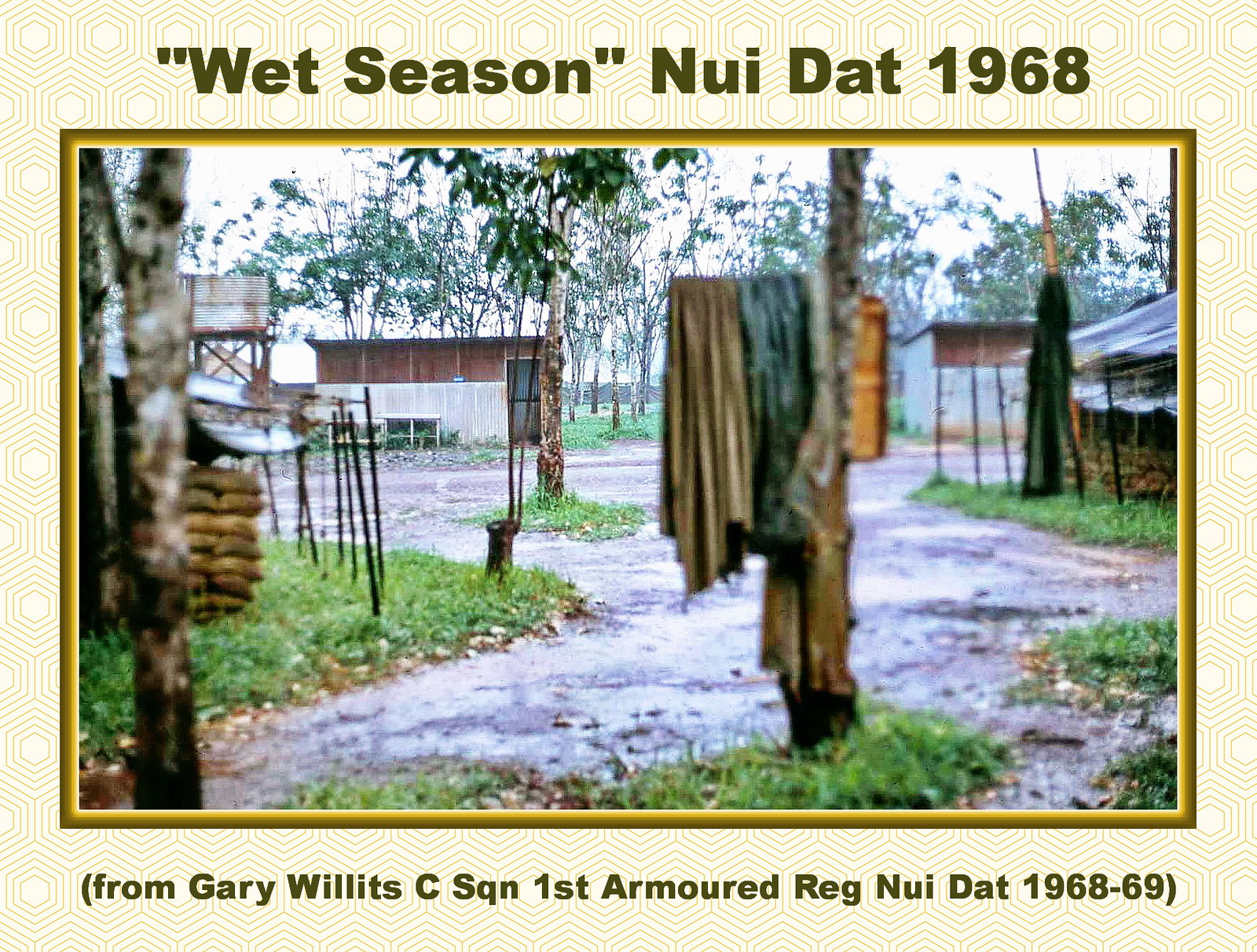This is a color photograph titled "Wet Season, Neu Dat, 1968" from Gary Willett's Sea Squadron, 1st Armored Reg, Neu Dat 1968-69. The image is presented in landscape orientation and features a rainy outdoor scene framed by a golden border adorned with a white and light gold hexagon pattern. The top of the frame bears the title in dark brown letters, "Wet Season," while the bottom reads, "Neu Dat, 1968."

The photograph captures a muddy pathway flanked by patches of grass and various structures. In the foreground, a tree trunk with a horizontal limb displays items of clothing, including brown and blue materials. This foreground is slightly out of focus compared to the remainder of the image. Besides the central path, there are several huts or shacks; one prominent structure on the right side rests on stilts and appears to be made of corrugated metal, with nearby sandbags forming a partial wall. In addition, the background features trees and a road that runs horizontally from right to left, enhancing the depth of the scene.